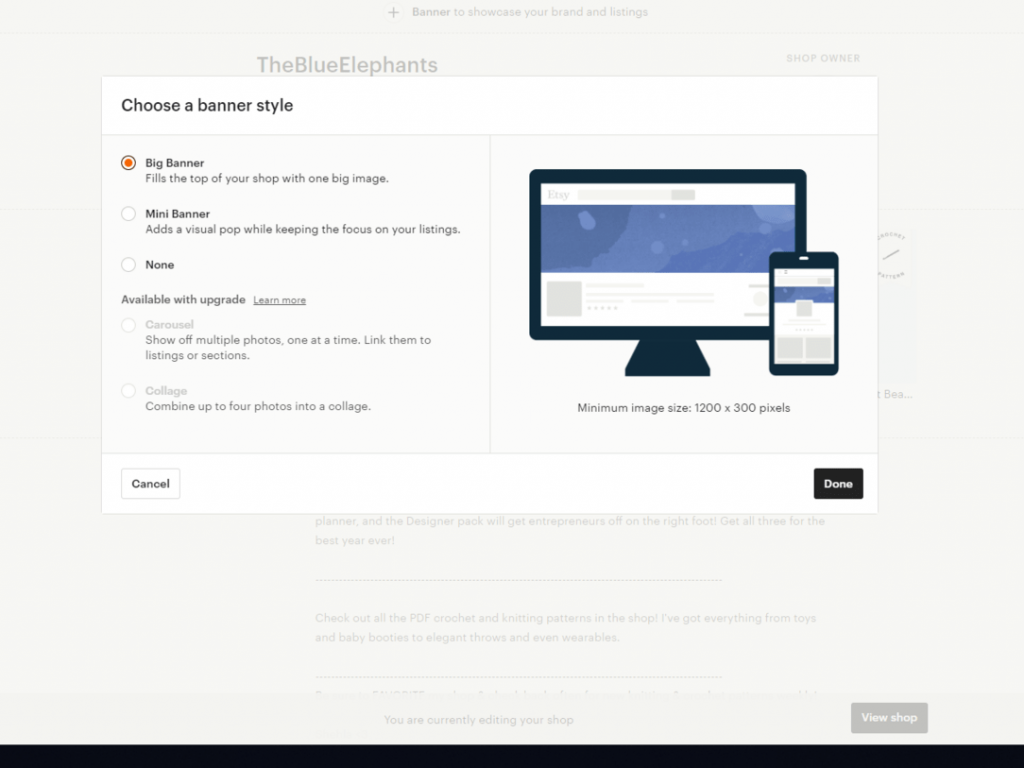Screenshot of a website interface featuring a page with a light gray background. In the center of the gray area, there’s a smaller white rectangle. At the top left of the gray background, the text "The Blue Elephants" is displayed. Inside the white rectangle, at its upper left, the heading "Choose a Banner Style" is presented, and beneath this, the option "Big Banner" is selected. A descriptive line follows: "Fills the top of your shop with one big image." 

On the right side of the white rectangle, an illustration depicts a black computer and a black cell phone. The computer, positioned slightly ahead, displays a screen with blue and white elements and blurred text. The cell phone, overlapping the computer on the right, shows a similar white screen with a blue bar across it. 

At the bottom of the white rectangle, on the left, a "Cancel" button is visible, and on the right, a "Done" button stands out in black with white text.